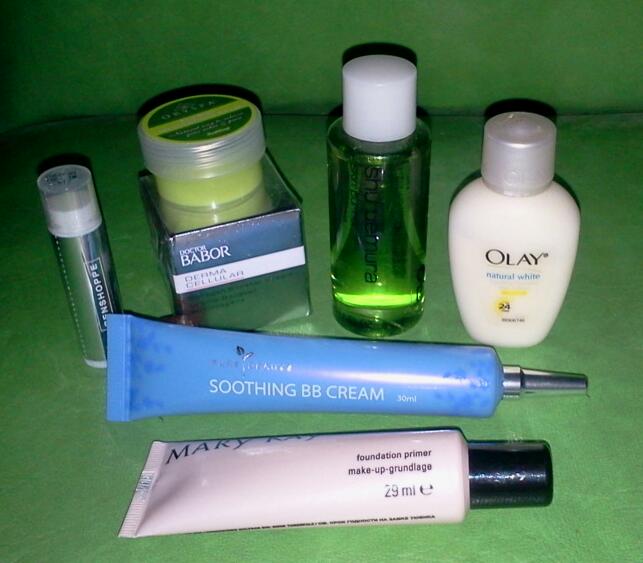The image showcases an assortment of six beauty products arranged on a green counter with a matching green background. From left to right, here is the detailed description of each product:

1. **Chapstick**: Positioned vertically on the far left, this green tube of chapstick does not display its brand or scent clearly.

2. **Dr. Babor**: Next to the chapstick, there is a silver box with a small, clear plastic container atop it. The container is filled with a yellow substance, has a green lid, and features yellow writing.

3. **Clear Plastic Tube**: Positioned to the right of the Dr. Babor item, this product is a clear tube containing a green substance and fitted with a white cap.

4. **Olay Natural White**: To the right of the clear tube, there is a white Olay bottle adorned with black letters that read "Olay Natural White." It is topped with a green cap.

5. **Soothing BB Cream**: Below the Olay bottle, a blue tube with white lettering declares it as "Soothing BB Cream."

6. **Mary Kay Foundation Primer**: The final product, positioned below the blue tube, is a Mary Kay foundation primer. The white bottle carries a black cap and specifies a volume of 29 milliliters.

The close-up arrangement of these items against a green setting gives a cohesive, color-coordinated appearance to the collection.